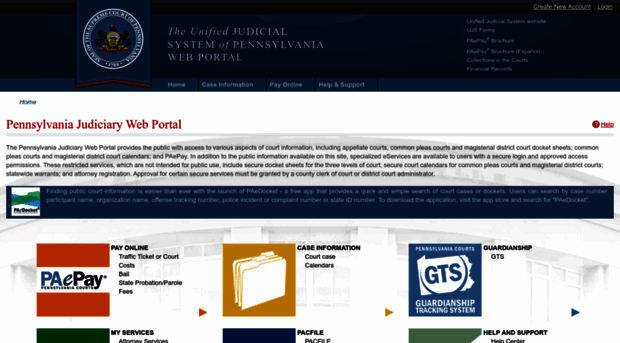This is a detailed screenshot of the Unified Judicial System of Pennsylvania web portal. At the top of the page is a dark blue banner featuring the state seal of Pennsylvania on the left side. To the right of the seal, there are several navigation links, though they are too small to be read in this image. In the extreme upper right corner, there are two buttons: one for creating a new account and another for logging in.

Central to the body of the webpage is a prominent title that reads "Pennsylvania Judiciary Web Portal." Below this header, there is a description outlining the website's purposes and functionalities, though the text is too small to be legible.

Towards the bottom of the page are three distinct boxes, each representing different functionalities of the portal. The leftmost box is labeled "PAePay," allowing users to pay bills online, presumably for Pennsylvania taxes and other state-related fees. The center box is titled "Case Information," providing a link for individuals to look up case details if they have an open case within the state. The rightmost box features an icon labeled "GTS" (Guardianship Tracking System), which is likely related to tracking and managing guardianship information though its specifics are unclear.

In summary, the web portal offers various online services including payment of state-related bills, case information lookup, and guardianship tracking, all organized within a clean and structured interface.